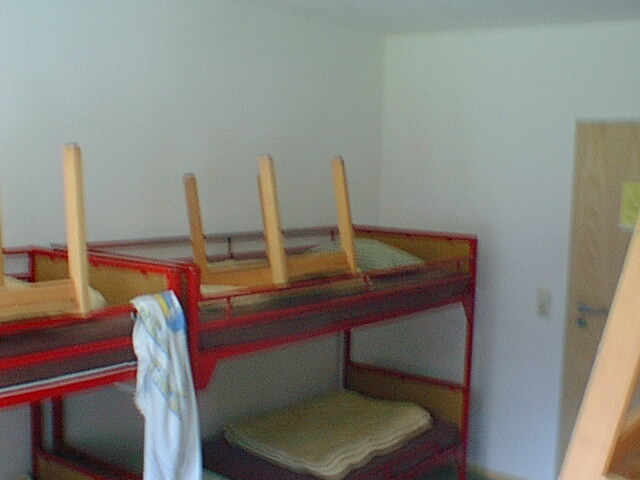The image depicts a blurry and low-quality photograph of what appears to be a dormitory or shared bedroom, possibly for small children. The photo is taken from the perspective of the top bunk, looking across to the opposite corner of the room. Visible in the room are at least two bunk beds made of red metal frames with purple mattress covers. Each bunk, both upper and lower, has neatly folded white blankets on the mattresses. A white shirt or towel is draped over the railing of one top bunk. Additionally, small square wooden tables have been placed upside down on the top bunks, possibly to clear the floor for cleaning. The room features pale white walls and a light brown wooden door with a yellow sign, the text of which is illegible. There also appears to be a ladder visible on the right side, suggesting an additional set of bunk beds. Overall, the image conveys a sense of tidiness and ongoing maintenance in the dormitory.